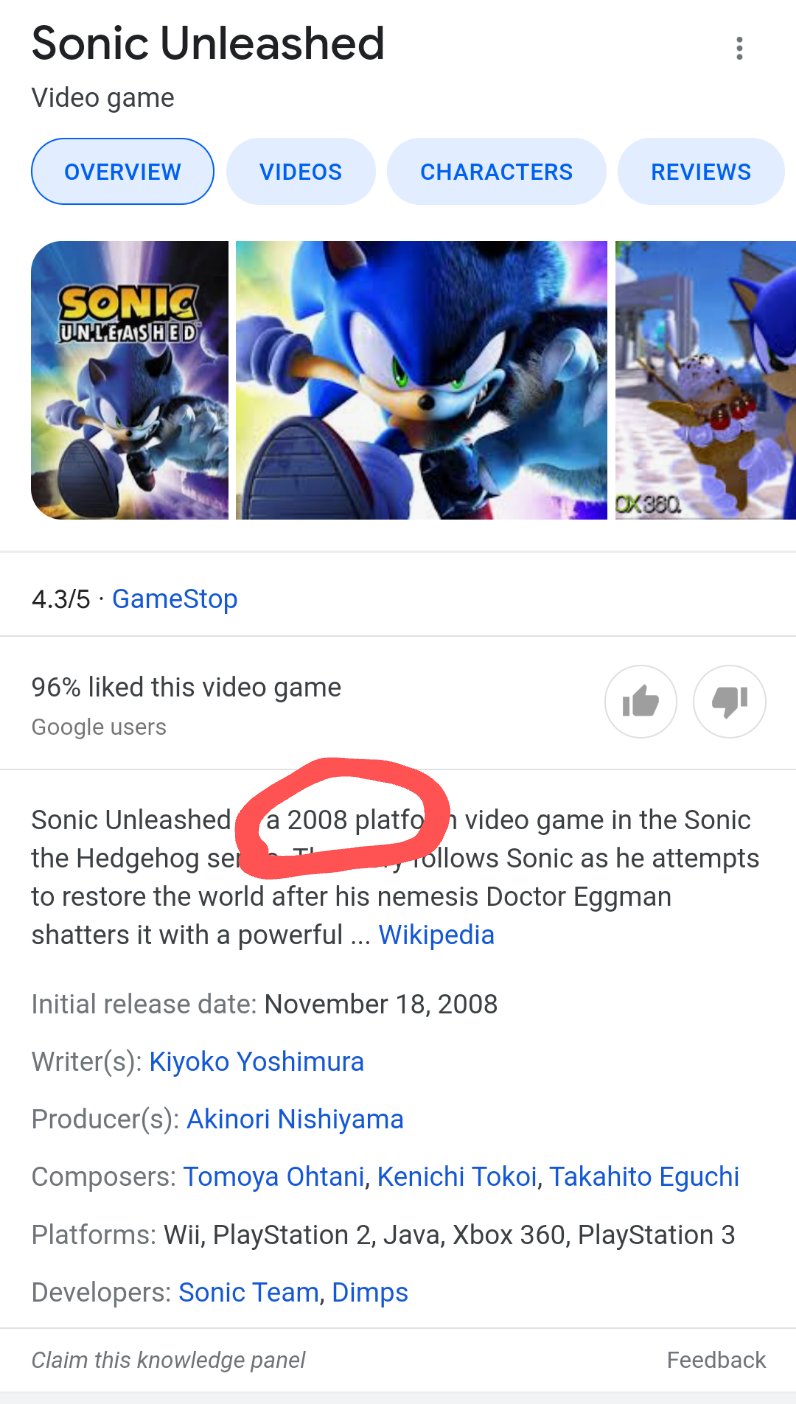A detailed screenshot captures an interface on a smartphone, specifically zoomed in on a search result for the "Sonic Unleashed" video game, viewed through Google. The rectangular shape and the large text on the screen suggest it is formatted for mobile viewing. The top of the interface displays several tabs, including "Overview," "Videos," "Characters," and "Reviews," with the "Overview" tab currently selected.

The distinct visuals in the overview tab showcase three photos from the game "Sonic Unleashed." The central image prominently features a modern 3D rendition of Sonic the Hedgehog, akin to the design seen in the recent movies. Sonic, in his signature blue color, is depicted running towards the viewer with an expressive and determined look.

Below the images, text highlights user ratings and reviews: Sonic Unleashed boasts a commendable 4.3 out of 5 rating on GameStop, and a striking 96% of Google users have expressed their liking for the game. Further down, a brief description, seemingly an excerpt from Wikipedia, provides context about the game. It states, "Sonic Unleashed, a 2008 platform video game in the Sonic the Hedgehog series, follows Sonic as he attempts to restore the world," although some of the text is truncated.

Overall, this screenshot not only provides a glimpse into the game's reception by users and critics alike, but also highlights key features and visuals that make "Sonic Unleashed" a notable entry in the Sonic the Hedgehog series.